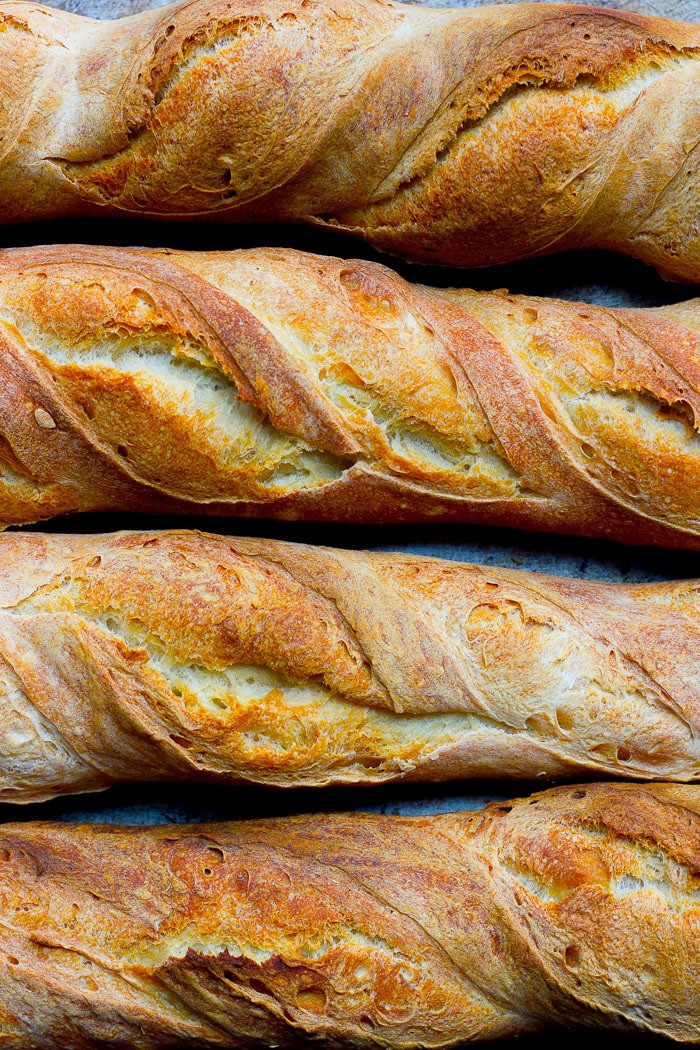The high-definition indoor image showcases four freshly baked French baguettes, stacked atop one another on a light gray stone countertop that barely peeks through beneath them. Exhibiting a beautiful browned crust with hints of lighter, almost cheesy yellow tones, the loaves appear irresistibly fresh, likely just pulled from the oven. The baguettes are long and thin, with a distinctive twisted pattern that has caused them to pop open in places, revealing their fluffy, white interior. Scores in the dough and a dusting of white powdery flour add to their artisan appearance, while the overall visual impression highlights their chewy, crunchy exteriors and soft insides.